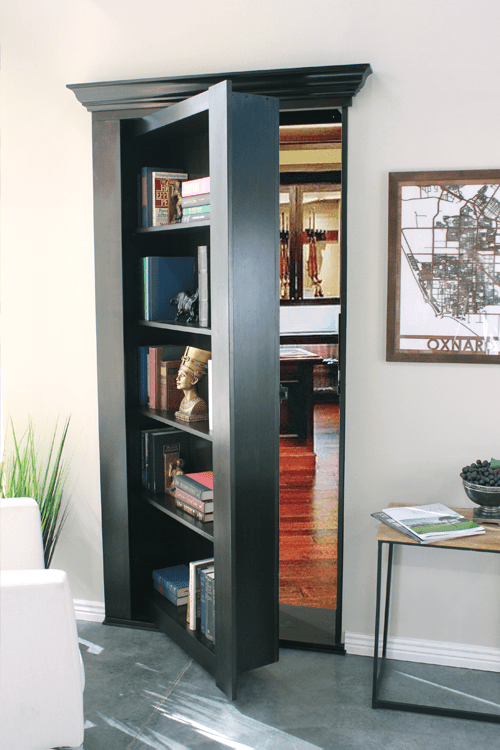This vertically oriented photograph captures the intriguing interior of a room with a cleverly hidden doorway. In the foreground, the room features a striking black bookcase set against white walls and a greyish-black marble floor. The bookcase, which serves as a hidden door, is slightly ajar, revealing another room behind it. This bookcase is adorned with approximately 20 to 30 books, an Egyptian statue reminiscent of Tutankhamun, and a few other figurines.

To the left of the bookcase stands a lush green floor plant, while to the right is a small desk with a magazine and a bowl that looks like it contains blueberries. Above this desk, a framed map of Oxnard in black, browns, and whites hangs on the wall. Nearby, a white chair contributes to the room's elegant yet functional decor.

Looking through the partially open bookcase, the hidden room behind reveals a warm, reddish-brown wooden floor contrasted against the cooler tones of the foreground. This secondary room includes a brown desk and what appears to be a display case, potentially containing firearms. Beige curtains with an orange and black design cover the windows at the back of this room, adding a softer touch to its mysterious allure. The hidden room's decorations add to the overall atmosphere, making it a fascinating focal point of the photograph. Additionally, the lighting throughout the entire space is bright and inviting, highlighting every intricate detail meticulously. A small, white object appears in the bottom left corner of the image, adding an element of curiosity to the composition.